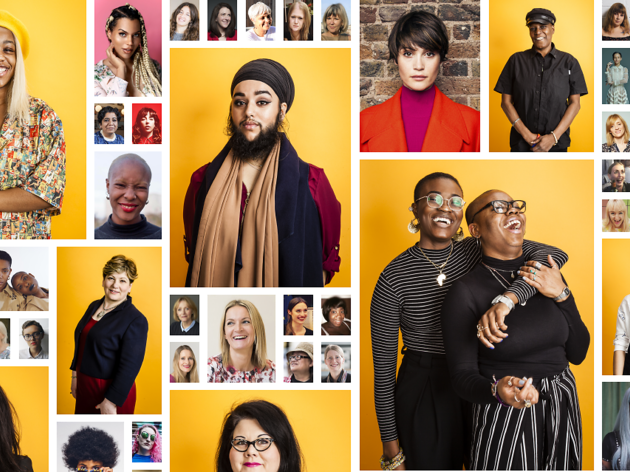This image showcases a collage of diverse portraits on a website likely dedicated to photography. The collage features a variety of headshots and full-body pictures, each differing in size and background color. The arrangement and style evoke the nostalgic feel of school photo exchanges, where friends would distribute and collect small prints.

Some portraits display bright yellow backgrounds, while others have varied settings, such as plain colored walls or a distinctive brick wall backdrop. One notable photograph features two Black women dressed in black, laughing together with one arm around the other, capturing a moment of shared joy. Another image against a brick background shows a white woman with short hair, wearing a red jacket over a pink shirt.

Among the collection, there is also an image of an individual with a beard and a large scarf, whose gender is not immediately clear. Most subjects in the portraits are smiling, adding to the overall warmth and friendliness of the collage. Another standout portrait features a woman with long hair set against a pink background. The majority of the images appear to be of women, with only a couple of individuals who might be men, but they too are likely women upon closer inspection.

In essence, this collage is a vibrant assembly of smiling faces and varied backgrounds, celebrating diversity and individuality.